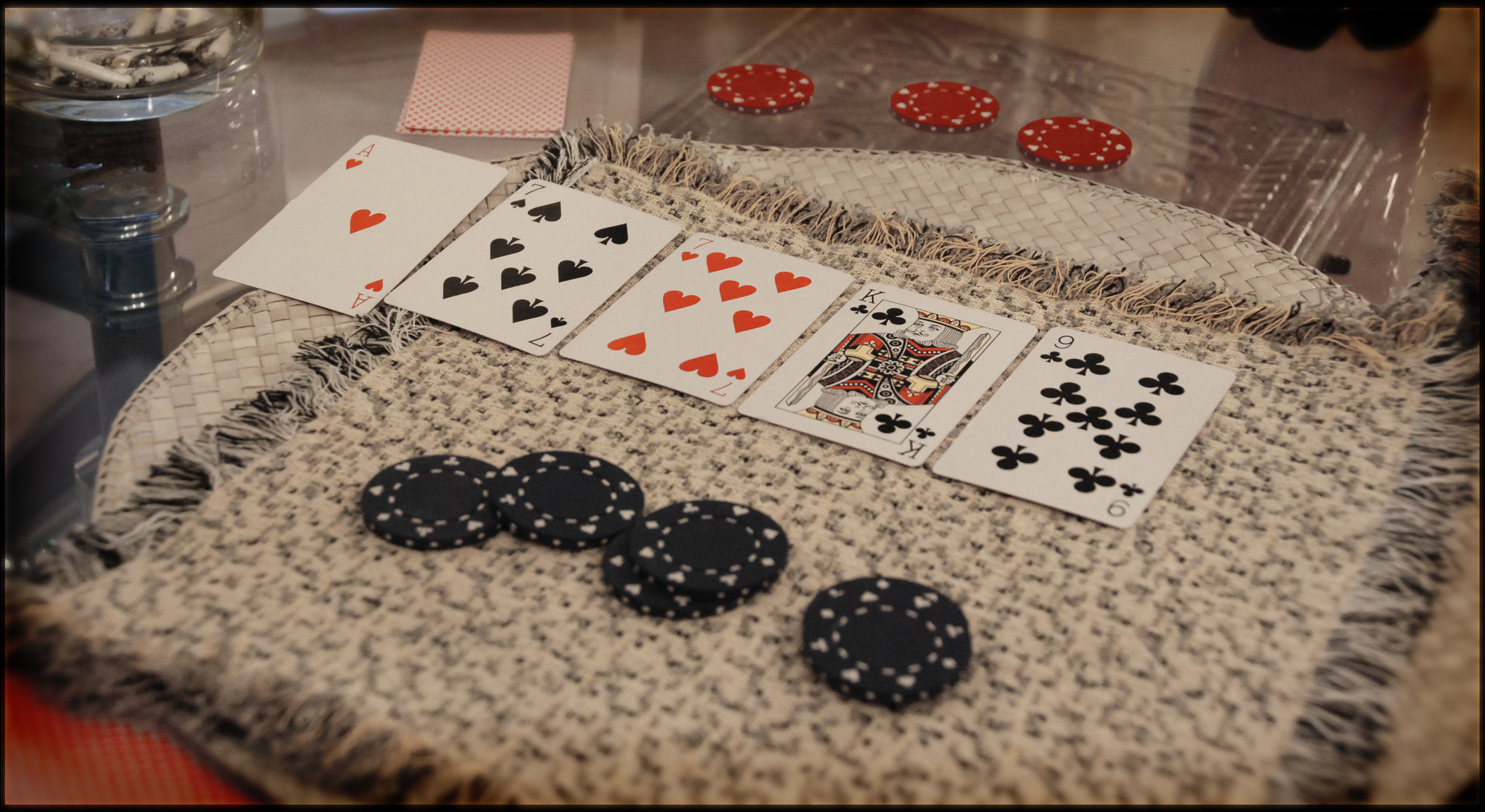A detailed photograph depicts a classic Texas Hold'em game setup. The central focus is on five playing cards arranged side-by-side from left to right: an Ace of Hearts, a Seven of Spades, a Seven of Hearts, a King of Clubs, and a Nine of Clubs. These cards rest on a cloth that is frayed around the edges, featuring a design of alternating black and light tan colors, all positioned on what appears to be a see-through glass table. 

Above the cards, three red casino chips are neatly stacked, while below them, four black chips are aligned. The chips are placed side by side, adding to the scene's organized chaos. The playing cards themselves are slightly tilted to the right at about a 45-degree angle, giving a dynamic feel to the arrangement. 

To the right of the Ace of Hearts, a clear, somewhat indistinct container can be seen, adding a touch of mystery to the photograph. The overall image captures the tense and intricate atmosphere of a poker game, with every detail meticulously laid out, from the frayed cloth to the precise angles of the cards.